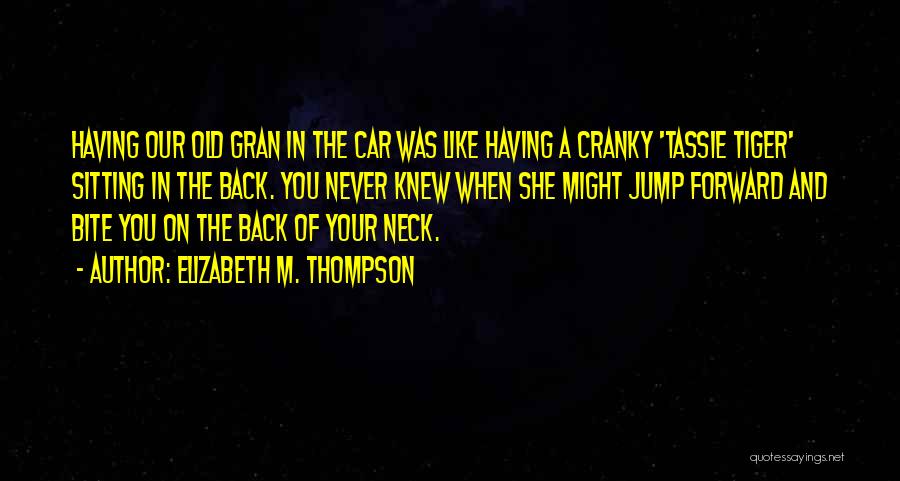The image features a plain black background with striking yellow text in a unique, horror-themed font that evokes a Halloween-like vibe. The text, written in all capital letters, reads: "Having our old gran in the car was like having a cranky, tassie tiger sitting in the back. You never knew when she might jump forward and bite you on the back of your neck." Beneath this quote is a credit line that reads "- Author: Elizabeth M. Thompson." In the bottom right-hand corner of the image, in white text, is the source "quotesayings.net," suggesting the image is designed as a motivational or inspirational quote, perhaps excerpted from one of Thompson's books.